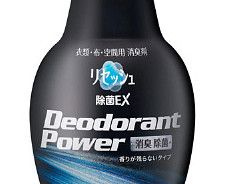The image depicts a black plastic bottle of deodorant powder situated against a crisp white background. The bottle, which has a curved, vertical oval shape with rounded edges, features the prominent white text "deodorant powder" centrally displayed. This text is flanked by rows of Asian characters, likely Chinese or Japanese, positioned both above and beneath it. A decorative element includes streaks or a chalky smear of blue and pale blue shades near the bottom of the container, adding a touch of visual interest. Additionally, some blue flowery imagery interspersed with Asian text can be seen at the top. The photograph appears to be a close-up, capturing only the middle section of the bottle with parts of the bottom and top cut off.